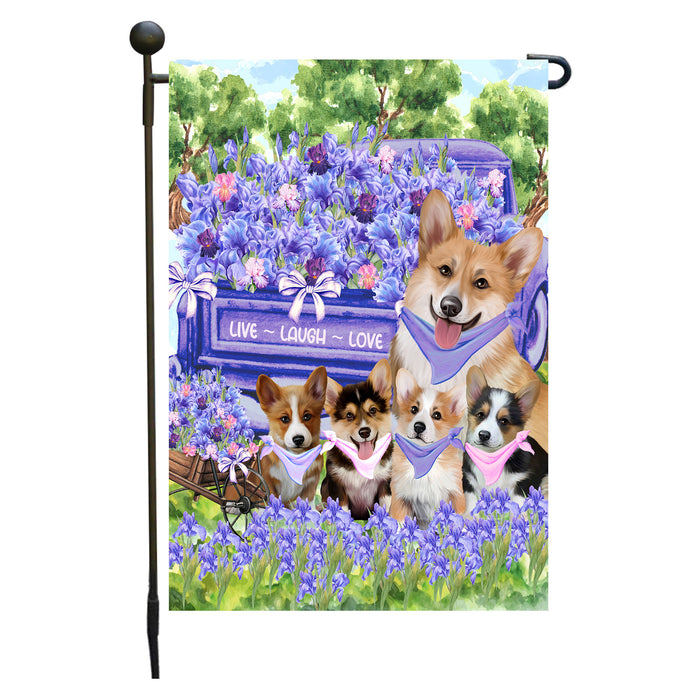The image features a decorative banner flag attached to a black flagpole with a rounded top and a hook extending to the right. The top of the banner showcases green trees against a light blue sky, with green grass below. The main focus of the banner is a vibrant display of mostly purple and pink flowers, paired with the depictions of five Welsh Corgi dogs, each donning either purple, pink, or white bandanas. The corgis, appearing happy with a mix of brown and black coats, are seated in front of a small purple truck filled with similar colored flowers. To the left of the dogs, there's a small illustrated wagon also adorned with flowers. Prominently written in white letters against a purple background are the words "Live, Laugh, Love," with a tied bow above, featuring a floral design to match the surroundings.